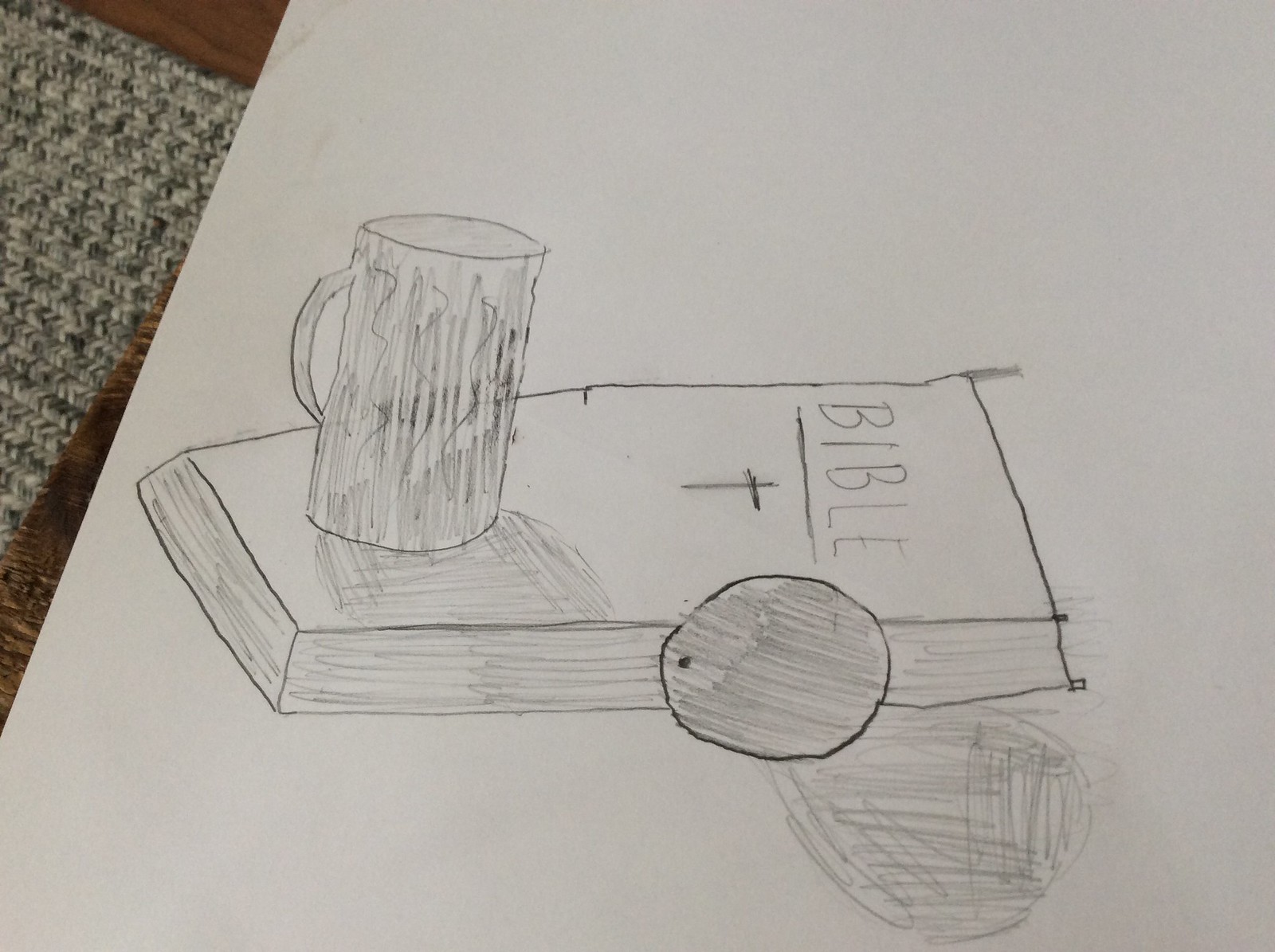The image depicts an indoor daytime scene with a juvenile pencil sketch on a large white sheet of paper. The sketch features a book labeled "BIBLE" in all capital letters with a cross beneath the title. A tall coffee mug, complete with a handle, is drawn atop the Bible, casting a shadow onto the book. Beside the mug is a round object resembling a piece of fruit, likely an orange, indicated by its spherical shape and a small dot at its base. The background reveals a fabric, possibly a green and white tablecloth or rug, partially covering a table. Above the rug, you can distinguish a portion of light to medium brown hardwood flooring. The overall impression is one of a simple, child-like drawing with notable details and shading.